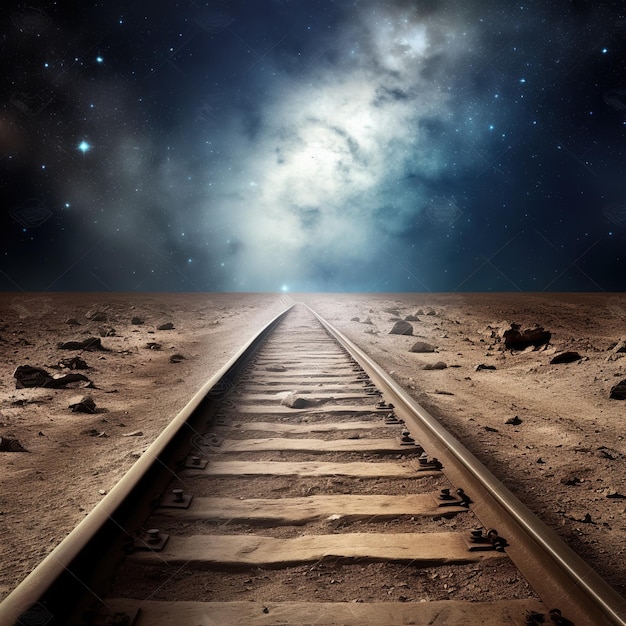The digital photograph presents a surreal juxtaposition: a solitary train track stretching into a barren, rocky expanse, gradually merging with the cosmos. The train tracks, devoid of any train, traverse the center of the image, bordered by brown dirt and scattered rocks. The overarching color palette comprises browns and tans for the earthen terrain, contrasted sharply by the deep blue and black hues of the sky. The sky itself is a mesmerizing canvas of space, adorned with countless stars and dominated by a luminous, blue-tinted cloud nebula at its center. This blend of terrestrial and astral elements, with no people or text, creates a hauntingly dreamlike scene, possibly alluding to a conceptual art piece or a fantastical rendition as might be seen in a digital game. The image is exceptionally clear, with distinct delineation between the desolate ground and the infinite celestial expanse, capturing the viewer's imagination as the tracks seem to lead directly into deep space.